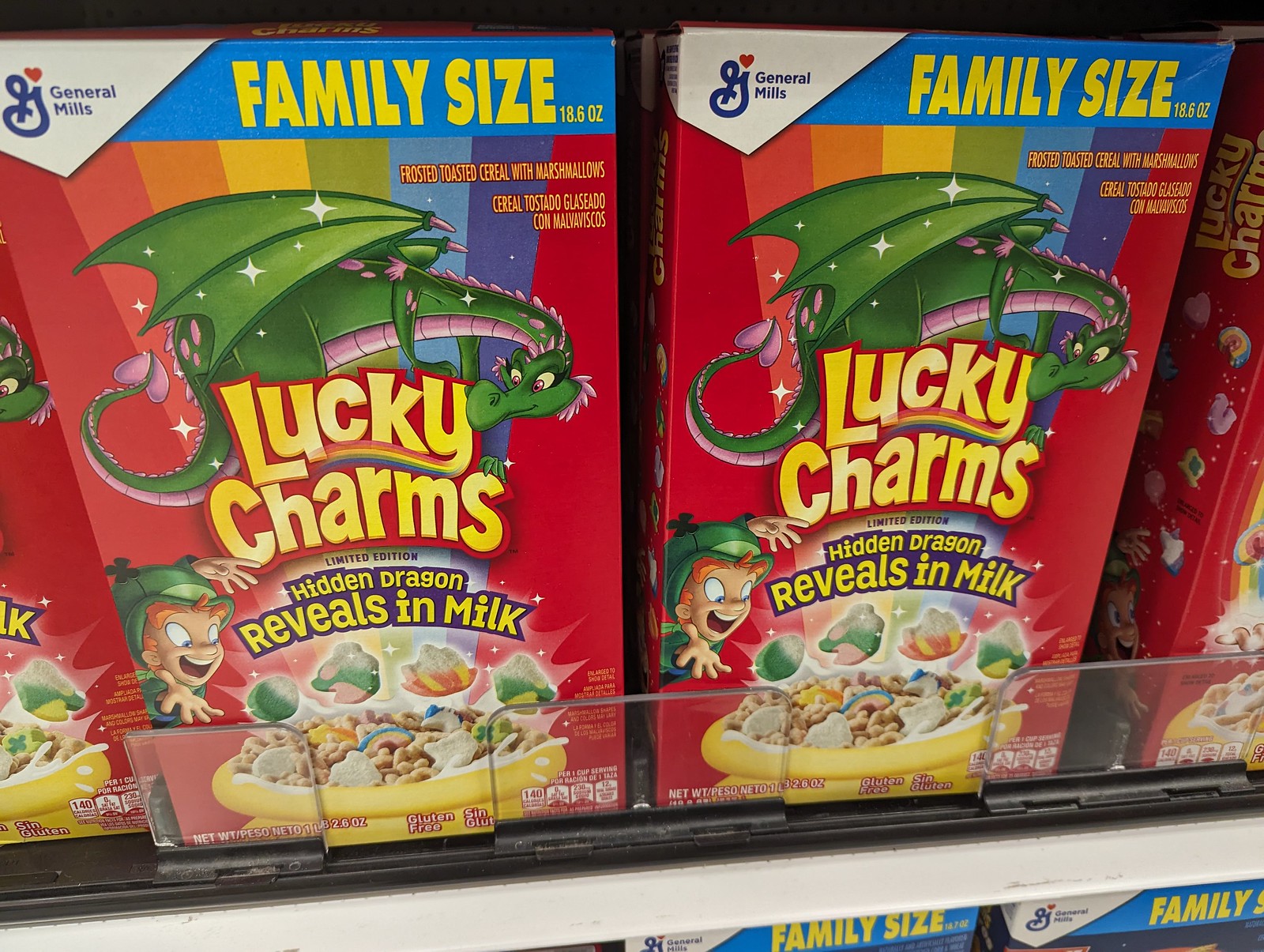The image captures a brightly lit grocery store shelf lined with vibrant boxes of family-sized Lucky Charms cereal. Dominating the scene are two fully visible boxes, with partial views of additional boxes flanking them on the left and right. Each box is predominantly red with a dynamic, colorful background featuring hues of orange, yellow, green, blue, and pink. Central to the design is a playful leprechaun gazing enticingly at a large yellow bowl of cereal filled with floating, multicolored marshmallows, seemingly tossing them in. Above this scene is a bold banner reading "Lucky Charms," partially enveloped by a majestically curling dragon, which is highlighted with pink accents. The text prominently advertises a "Limited Edition Hidden Dragon Reveals in Milk." The top of the box sports a blue banner with "Family Size" written in bright yellow, accompanied by the General Mills logo on the top left. The overall aesthetic is meant to entice shoppers with its magical and whimsical design.